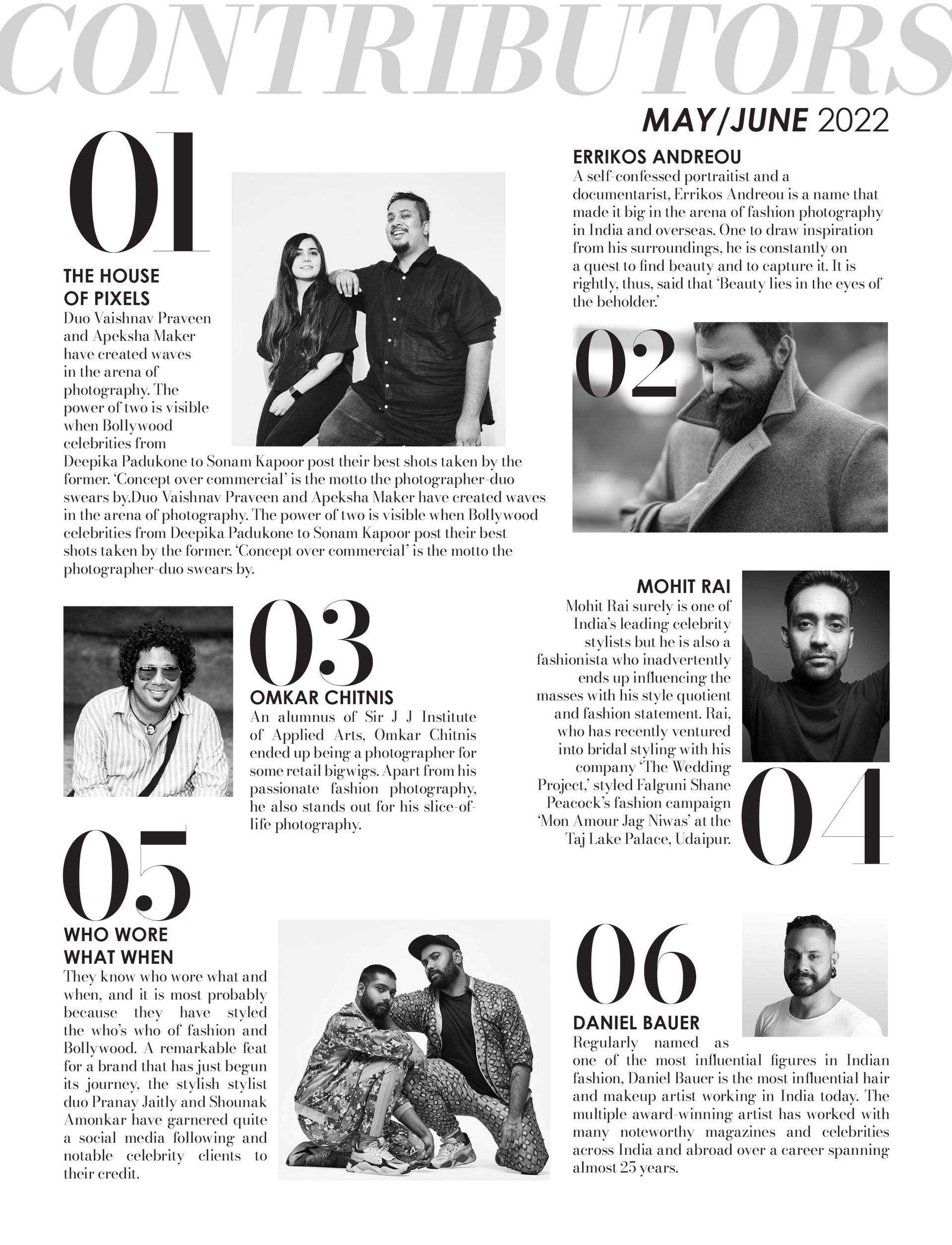The black and white magazine page, labeled "Contributors, May/June 2022," prominently features six contributors, each with an accompanying photograph. The contributors are numbered in bold black font:

1. The House of Pixels: A photo of duo Vashnav Praveen and Apeksha Maker, known for their impactful photography, particularly of Bollywood celebrities like Deepika Padukone and Sonam Kapoor. Their motto, "Concept over Commercial," underscores their creative ethos.
   
2. Erica's Andrew: A man posed in a coat, contributing his expertise to the magazine's content. 
   
3. Omkar Chitnis: Pictured in a long-sleeved striped shirt and shades, adding his unique style and perspective.
   
4. Mohit Rai: Shown in a black turtleneck, providing his insights and likely fashion expertise.
   
5. Who Wore What When: Featuring two men dressed in coordinated printed outfits, including jackets, pants, and caps, showcasing fashion trends and styles.
   
6. Daniel Bauer: Depicted in a t-shirt with his hair plaited back, contributing his knowledge and skills to the edition.

This page, with its structured layout and black and white theme, introduces the diverse and talented contributors of this magazine issue.